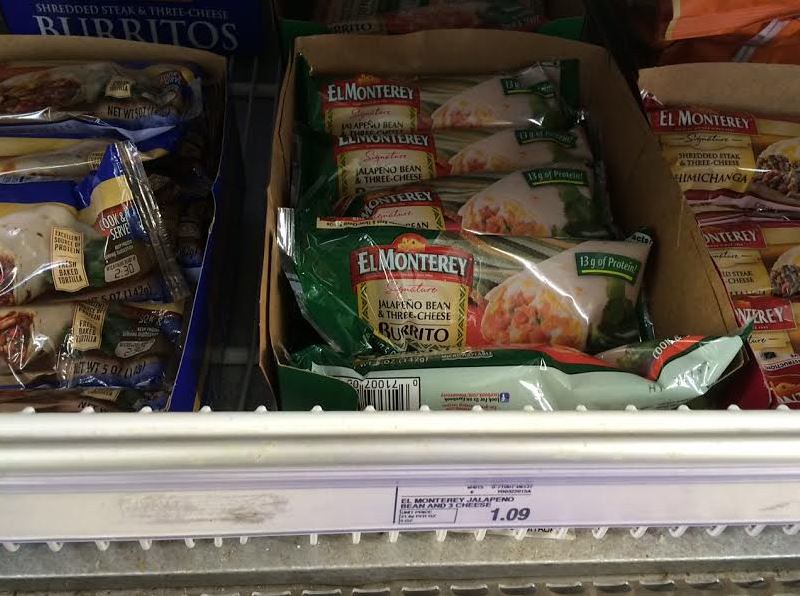This photo was taken inside the freezer section of a grocery store. At the center of the image is a box of El Monterey Signature Jalapeño Bean & Three Cheese Burritos, distinguished by its green and white packaging. The box, which contains five burritos, features a picture of an appetizing burrito on the front. A black and white price sticker in front of the freezer indicates that each box costs $1.09. Surrounding this focal box are other El Monterey products, including the Chimichanga variety, neatly stacked on the shelves. The attention to detail and emphasis on the green burrito box highlights its prominence among the other frozen selections.